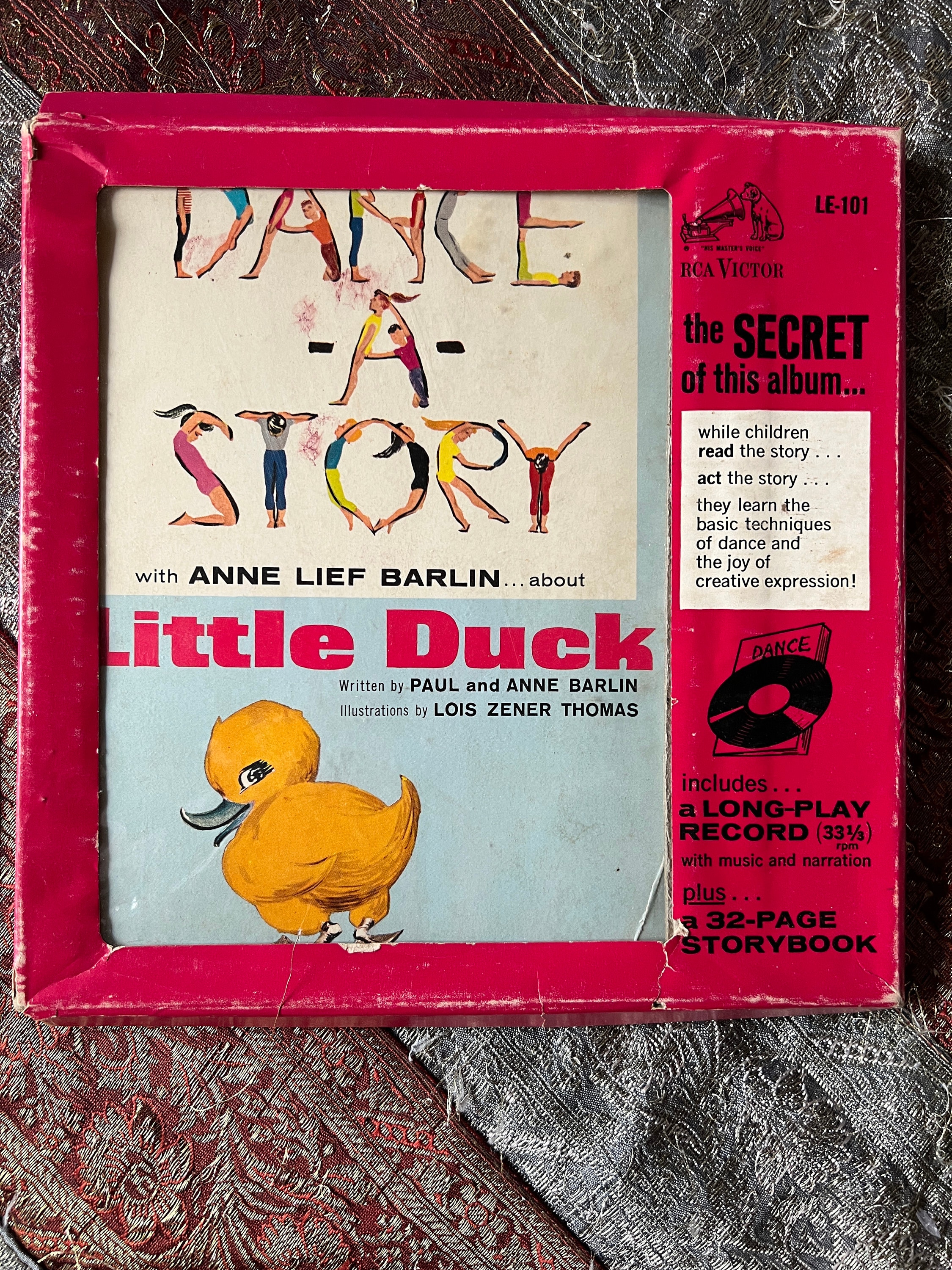The image depicts a vivid and intricately designed red cardboard box. At the center of the box is a square cutout revealing the words "Dance A Story," each letter creatively formed by animated cartoon characters in various dance poses. Beneath this playful title, it reads "with Anne Leif Barlin" and "Little Duck" in dark red font. Further below, it states "written by Paul and Anne Barlin" and "illustrations by Lois Zinner Thomas." The illustration features an endearing, fluffy yellow duckling with a gray bill, positioned to appear as if turning its head to look directly at the viewer. 

On the right side of the box cover, the text "The Secret of this Album" is visible. Below this, a description in black font on a white background reads: "While children read the story, act the story, they learn the basic techniques of dance and the joy of creative expression!" Included is a depiction of the album, accompanied by a booklet titled "Dance," explaining it includes a "long-play record 33 1/3 with music and narration" and a "32-page storybook." This scene is meticulously placed on a fancy tablecloth, adding to the overall charm and detail of the presentation.